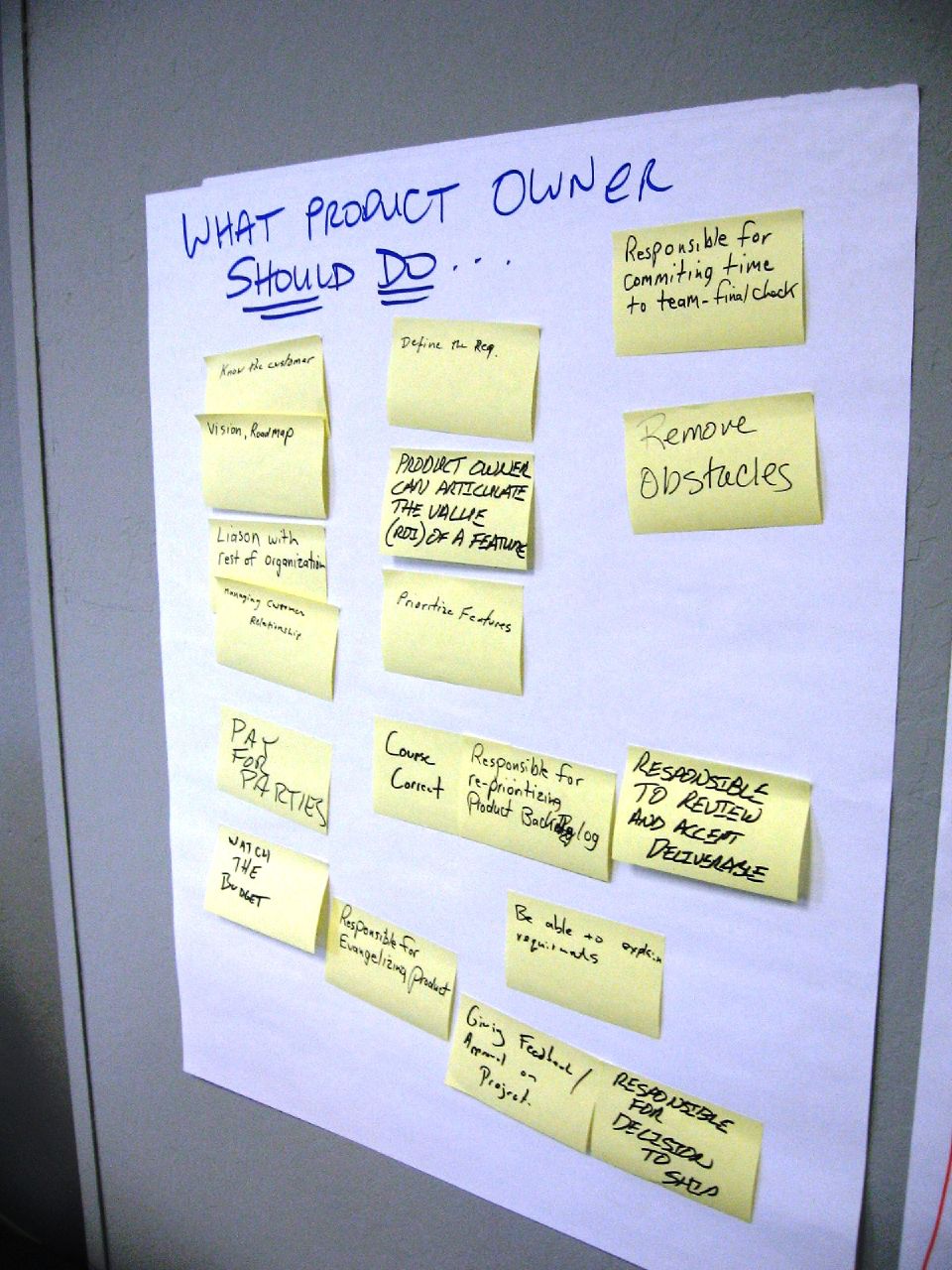The image captures an office setting with gray walls and features a large sheet of white paper taped to the wall, which appears to be part of a brainstorming session. The paper, titled "What Product Owners Should Do," is written in blue font with the words "should do" underlined twice. Below the title, there are approximately 15 to 20 sticky notes arranged in three slightly skewed columns. 

In the first column, there are six sticky notes. The second column has five sticky notes, with three additional notes positioned toward the bottom, separate from the rest. The third column on the right contains four sticky notes. The writing on the notes varies in clarity, with some entries being more legible than others. Notable examples include directives like "watch the budget," "pay for parties," "remove obstacles," "responsible for committing time to team," "responsible to review and accept," "course correct," "giving feedback," and "appeal on project." The collection of notes suggests this was an interactive session, possibly involving students or employees, aimed at outlining the essential responsibilities of a product owner.